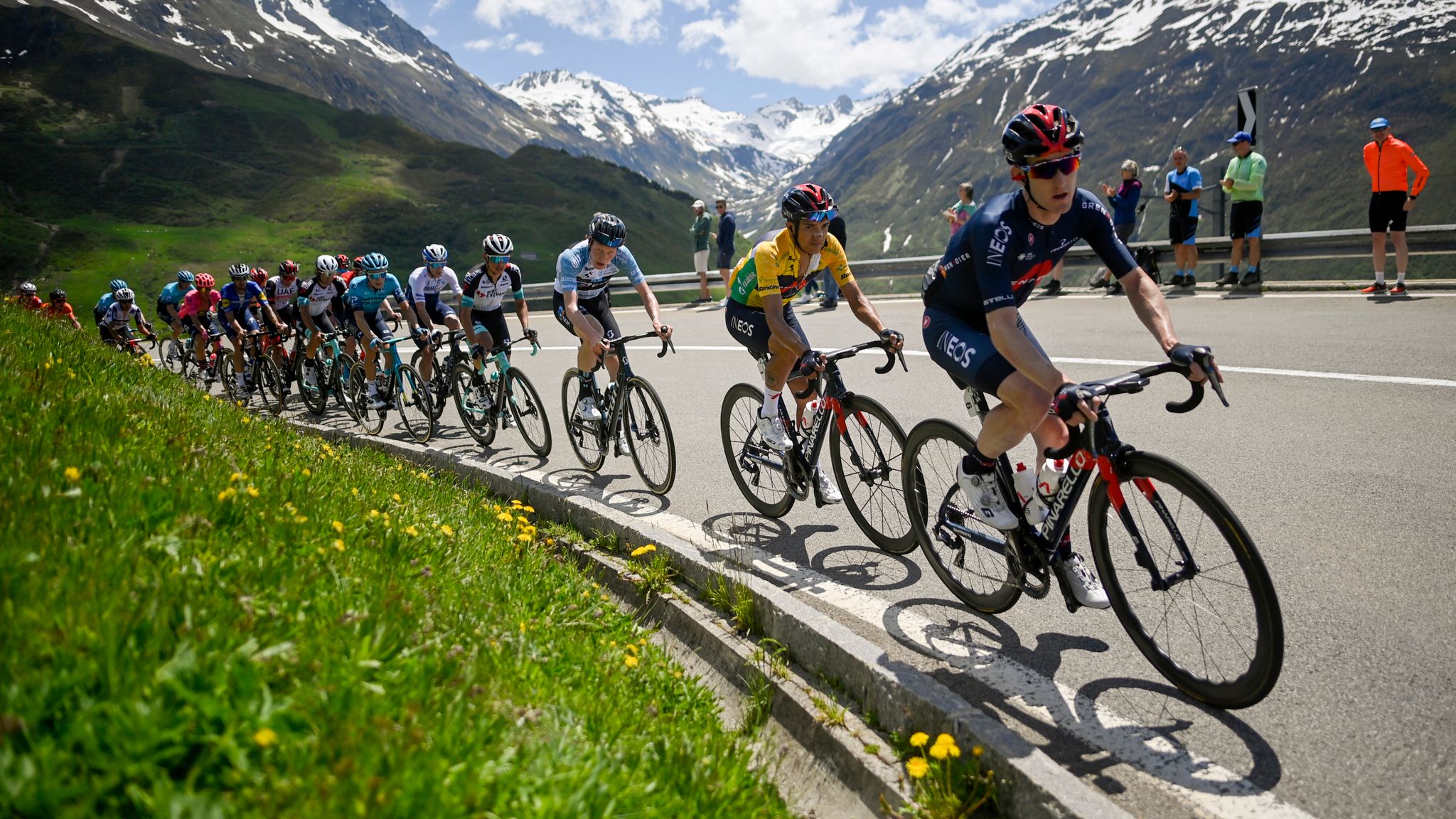In this vertical photographic image set in a mountainous outdoor location, a group of cyclists, possibly competing in a prestigious race such as the Tour de France, are navigating a winding road with gray asphalt and a white stripe near the curb. The leading rider is donned in a red and blue helmet, a blue and white jersey, black pants labeled "EOS," and sunglasses, riding a black and red bicycle. Directly behind him is a cyclist with similar black pants labeled "EOS," wearing a yellow and green jersey and the identical red and blue helmet, also riding a black and red bicycle. The second cyclist appears to be of Hispanic or South Asian descent, while the first and third cyclists, who wears a blue and white jersey similar to the lead rider, are white. Following them is a sequence of riders in various colored jerseys – a black and white jersey, a white jersey, and a blue jersey, among others. They ride in a disciplined line along a curve that heads to the bottom right of the image.

On the right side of the road, a group of approximately eight spectators observe the race, standing by a guardrail. They are dressed in a mix of casual summer attire: shorts and a variety of shirt colors, including orange, green, blue, and black, with a few wearing black baseball caps. Some spectators appear to be clapping, adding to the dynamic atmosphere of the race. The backdrop features a stunning range of snow-capped mountains under a clear blue sky, and the immediate roadside is adorned with patches of green grass and clusters of small yellow flowers, possibly dandelions. This picturesque mountainous setting, reminiscent of the Swiss Alps or the Rockies, adds a breathtaking scenic element to the intense cycling competition.